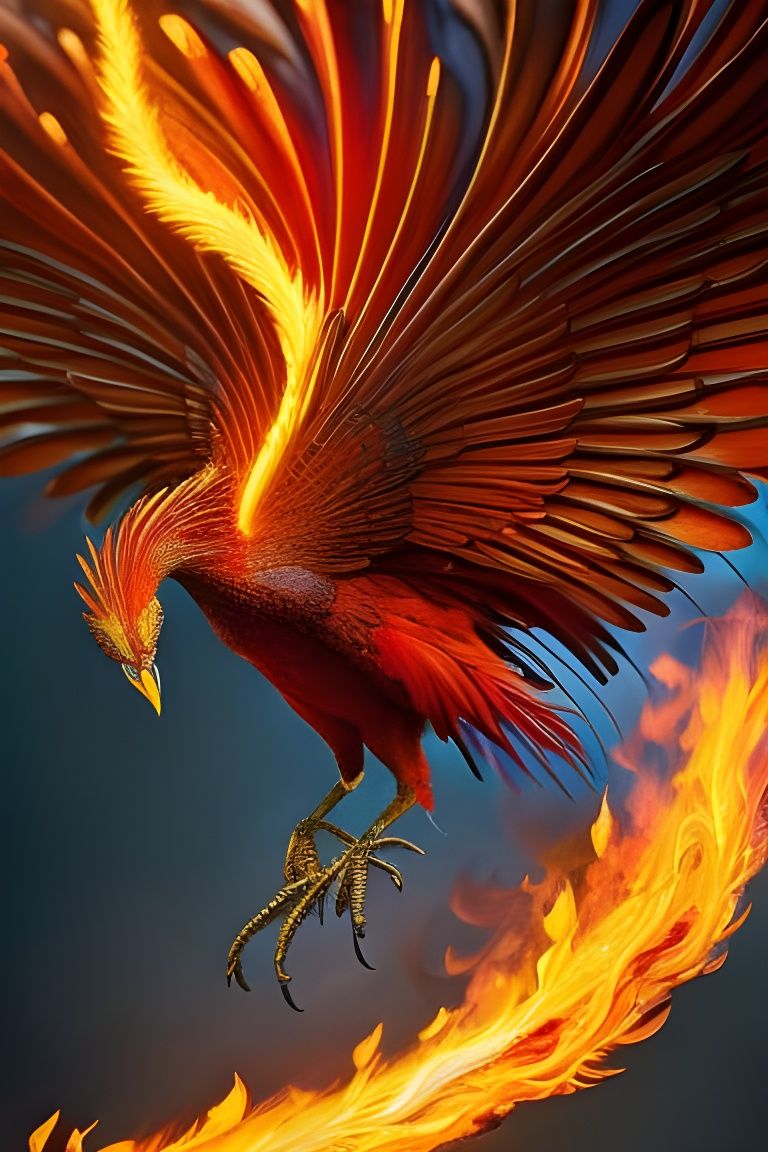This detailed illustration features a majestic phoenix, radiating vibrant colors against a varying shades of blue background. The phoenix's feathers are primarily a fiery red with accents of yellow, giving the impression of an otherworldly glow. Its yellow beak stands out, and the eyes, a striking blue, are fixed in a downward, backward gaze. The bird is depicted mid-flight, wings fully extended with long, vivid feathers. Prominent claws, brown and talon-like, reach downwards, adding to the dynamic sense of motion.

A mesmerizing interplay of flames surrounds the phoenix, enhancing its mythical aura. Golden-yellow flames arc upwards from behind the bird, shimmering and illuminating its wings. Below, an intense burst of orange, yellow, and red flames suggests the phoenix's legendary rise from the ashes. The flames merge seamlessly with the phoenix's body, reinforcing its ethereal rebirth. This detailed, vibrantly colored graphic captures the essence of the phoenix amid its fiery, symbolic ascent.